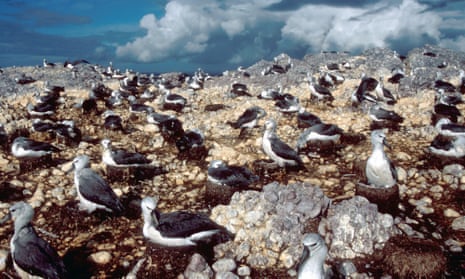This is a color photograph depicting a rocky shoreline populated by a large number of seabirds, approximately around 50 to 60, scattered across the gray and beige rocks. The photograph is somewhat blurry, making it challenging to precisely identify the species. The birds are characterized by their white heads and breasts, and dark gray or black backs. They have dark beaks and a size comparable to that of pigeons. The backdrop features a dark blue, stormy sky with thick, billowing clouds, suggesting an overcast day with no visible sun, adding to the moody atmosphere. The foreground appears to have darker, possibly damp soil, hinting at the proximity to water. No other animals, people, buildings, or mechanical objects are present in the image.